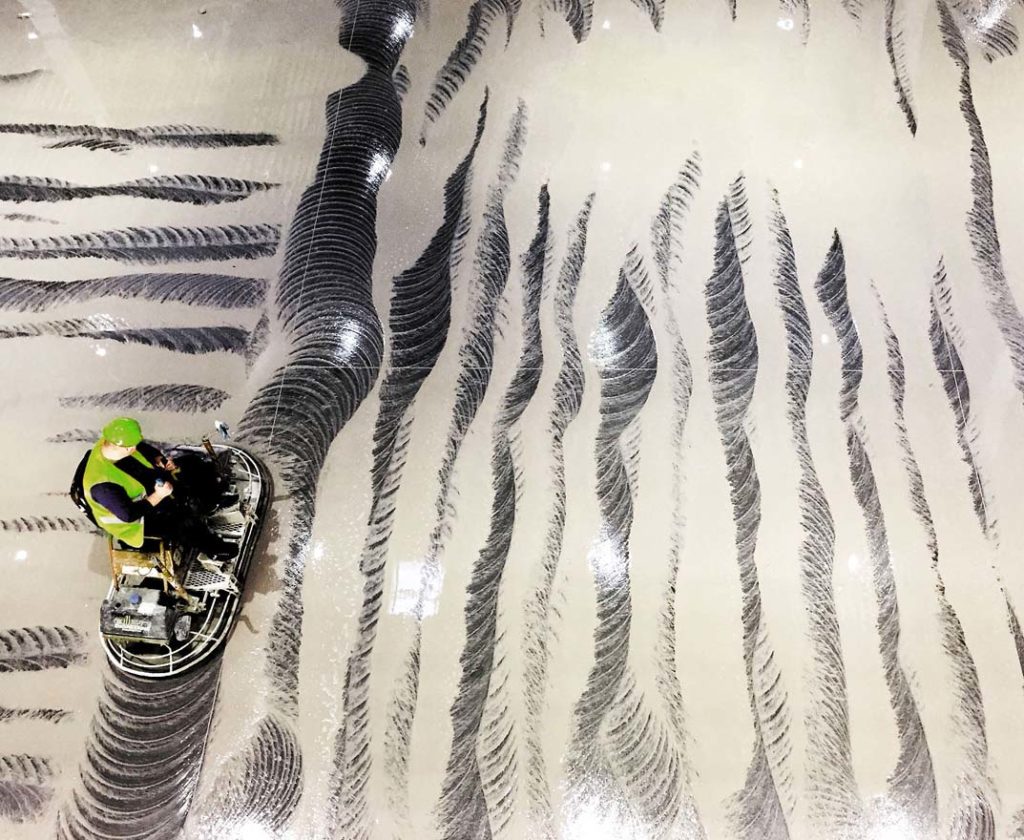In this photograph, we see an aerial view of a large, tan-colored floor that glistens with a marble-like sheen. The texture of the floor is interrupted by a series of undulating, black squiggly lines, reminiscent of a zebra pattern or perhaps brush strokes. The lines suggest movement and might be intentional markings or a byproduct of some process. On the lower left corner of the image, a construction worker is visible, seated atop an oval, pill-shaped piece of machinery. The worker is wearing a lime green hard hat and matching vest, with the rest of his attire being black. The machinery he operates is surrounded by a white cage-like frame and appears to have rotors or vents on its sides. The worker uses two joysticks to maneuver the machine, which could be either polishing or painting the floor, as it leaves those distinct black marks behind. The function of the machine, while uncertain, is clearly central to the creation of the patterned lines on the floor.